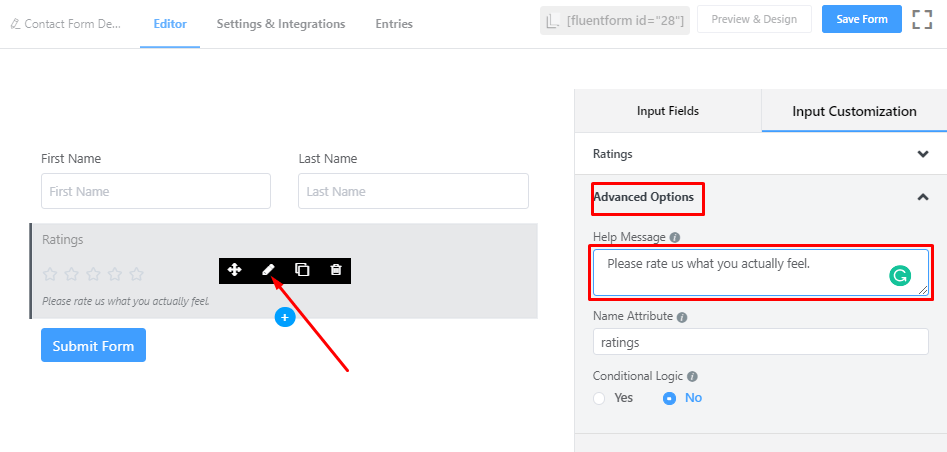On this web page, with a clean white background, the top navigation bar features several elements arranged from left to right: a contact form icon, a "DE..." dropdown menu, and tabs labeled "Editor," "Settings," "Integrations," and "Entries." On the far right of this navigation bar, there is a gray button displaying the text "Fluent Form ID = '28'," a white "Preview and Design" button, and a prominent bright blue "Save Form" button with white text.

Beneath the navigation bar, a thin gray line spans the width of the page, serving as a subtle separator. Within the navigation, the "Editor" tab is currently selected, highlighted in bright blue with an underline for emphasis.

The main content area, also set against a white background, begins with two text input fields: one labeled "First Name" on the left and another labeled "Last Name" on the right. Below these fields, there is a light gray horizontal box titled "Ratings," featuring five stars for user rating. Underneath the stars, in small italicized text, it reads, "Please Rate Us What You Actually Feel." 

Adjacent to the rating section, a black box contains a long red arrow pointing towards an edit icon, which resembles a small pencil. At the bottom of this form, a bright blue "Submit Form" button with white text stands out, ready for users to finalize their input. Additional content is visible on the right side of the page, though it is not detailed in this description.